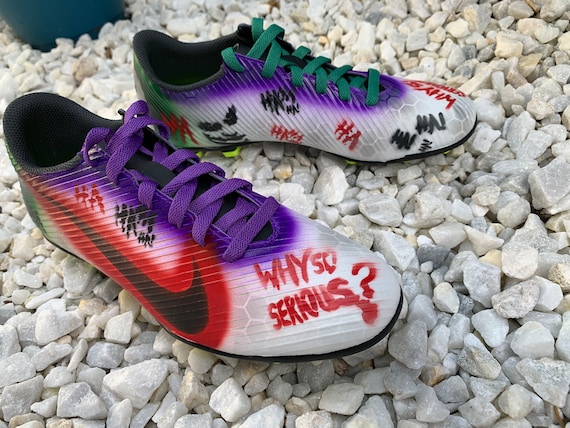The image shows a pair of custom-designed cleats for soccer, football, or baseball, displayed on a bed of white gravel. Each shoe features a Nike logo, highlighted in black against a red background. Across both shoes, "ha, ha, ha, ha" is handwritten in vibrant black and red, along with the iconic phrase "Why so serious?" imprinted on the toe areas in bold red letters. The laces are mismatched and striking—one shoe has deep blue laces that verge on purple, while the other has green laces. The cleats also incorporate a stylized face with eyes, a nose, and a mouth, complementing their Joker-themed design. These unique, Joker-styled cleats offer a playful yet eerie vibe, perfect for standing out on the field.